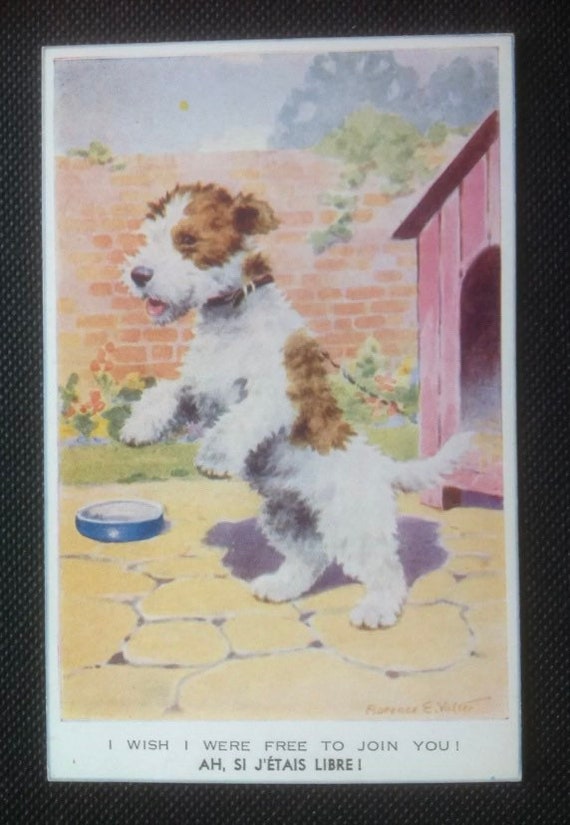In a vertical rectangular frame sits a vibrant watercolor illustration on a white piece of paper, bordered by black and gray speckles. The artwork, reminiscent of a comic panel, captures a small, white dog with brown spots and ears, and a black nose. The dog, looking somewhat unkempt yet content, is depicted standing on its hind legs as if wanting to break free from the chain and collar that tethers it to a pink wooden doghouse on the right. To the dog's left, a blue food bowl rests on a patio made of paving stones. The background features a red brick wall adorned with small green, red, and yellow flowering bushes. Below the illustration, in black text, it reads, "I wish I were free to join you," with an additional phrase in French underneath.